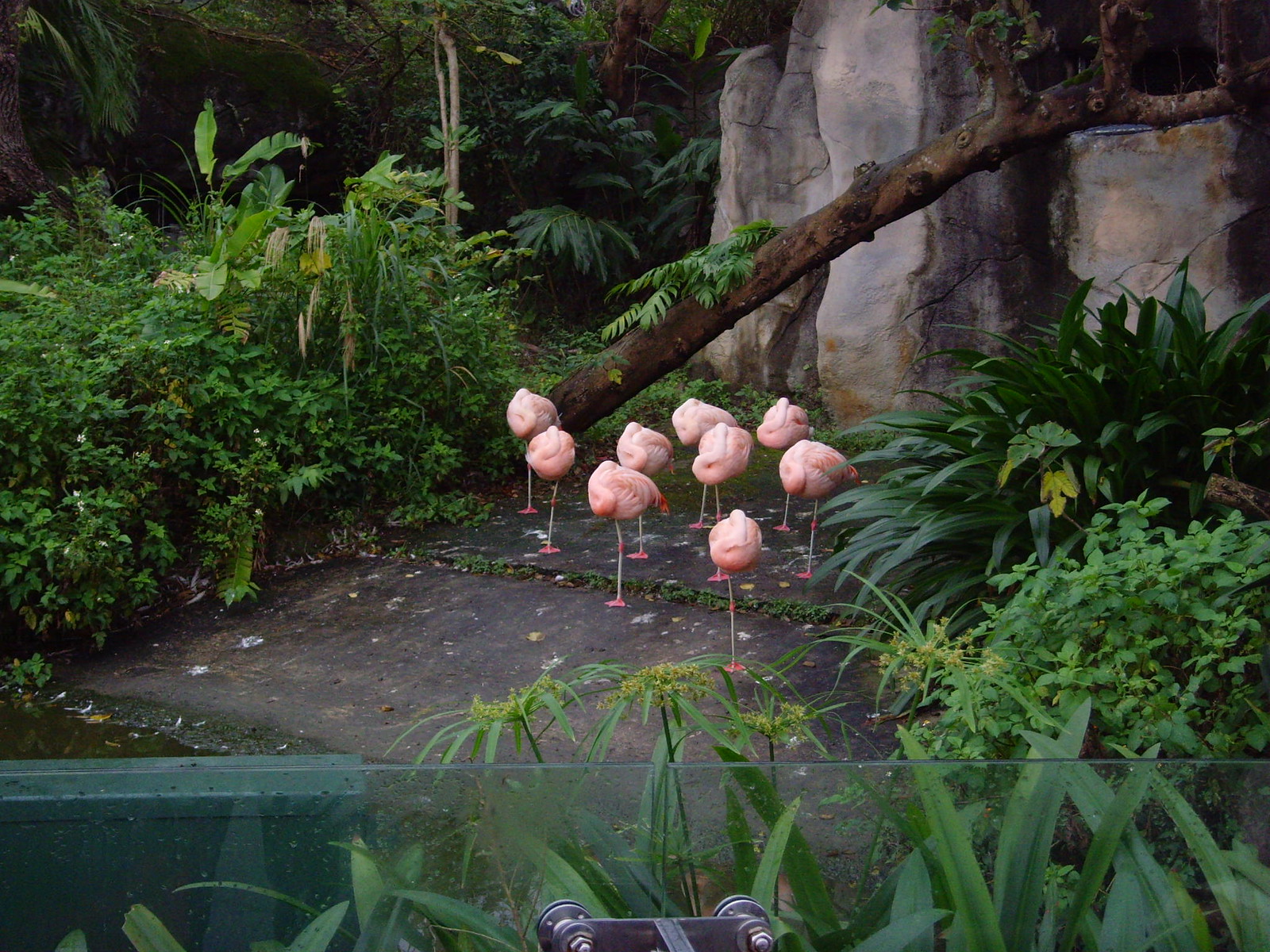This vibrant color photograph captures a serene scene featuring a cluster of nine pink flamingos, predominantly standing on one leg with their heads tucked back over their bodies, suggesting they are sleeping. Centered in the image, these flamingos rest on flat rocks and brown dirt, surrounded by lush, verdant foliage. In the background, a large boulder rises, complemented by a fallen wooden log that extends diagonally from the boulder’s base up towards the right edge of the frame. Enhancing the sense of enclosure, a clear glass divider with a metal apparatus at the bottom is visible in the foreground, creating a boundary between the viewer and the tranquil, natural habitat.